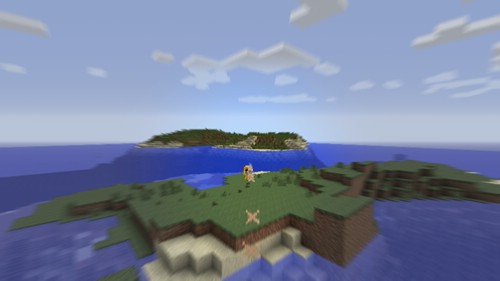The image is a detailed screenshot from the game Minecraft. In the background, a clear blue sky with fluffy white clouds stretches above a large body of shimmering water, reflecting portions of the scenery. In the middle distance, a mountainous area peaks into view, its rocky terrain speckled with green foliage, presenting a mix of brown earth and lush greenery. In the foreground, an island made of irregularly shaped green blocks, underlaid with brown dirt, stands prominently. At the very bottom corner, a light tan block area forms the base, while a small figure, presumably a game avatar, is discernible in the center of the green expanse. Additionally, a distinct yellow X-marked block appears in the lower portion of the scene, adding to the structured, pixelated landscape definitive of Minecraft.